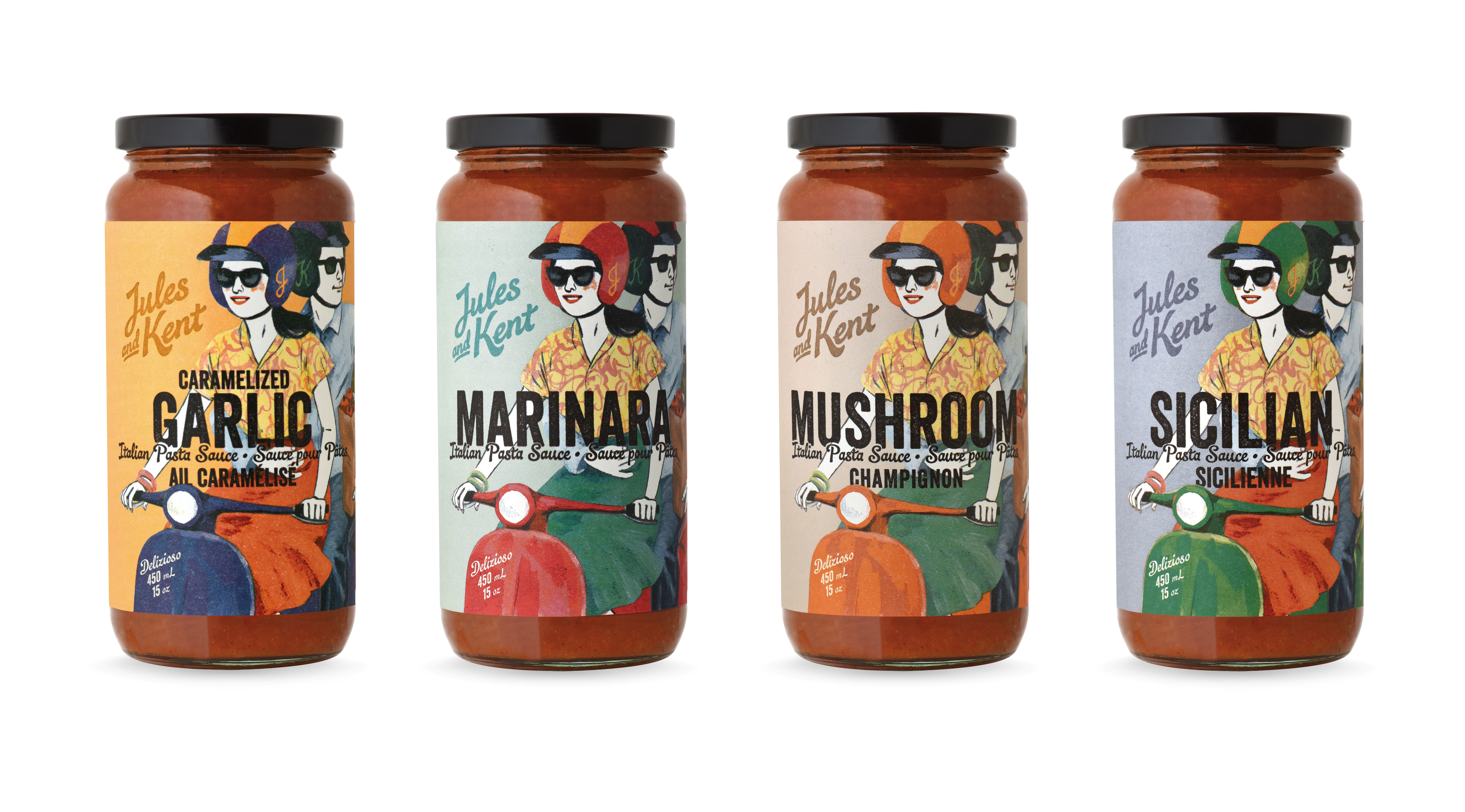This image features four jars of Italian pasta sauce, each from the brand Jules and Kent, arranged horizontally against a white background. Distinctive black lids top the full glass jars, each containing a rich, red pasta sauce. The first jar is labeled "Caramelized Garlic," followed by "Marinara," "Mushroom," and "Sicilian." All jars share a whimsical, cartoon-like illustration depicting a man and woman on a moped, with the man seated behind the woman, his arm wrapped around her waist, while she handles the handlebars. Their helmets, the moped, and the background colors vary for each sauce flavor - blue for Caramelized Garlic, red for Marinara, orange for Mushroom, and green for Sicilian - adding vibrant, playful details to the packaging. Each label also prominently displays the brand name Jules and Kent in the upper left corner, emphasizing the colorful, animated theme across all variations.